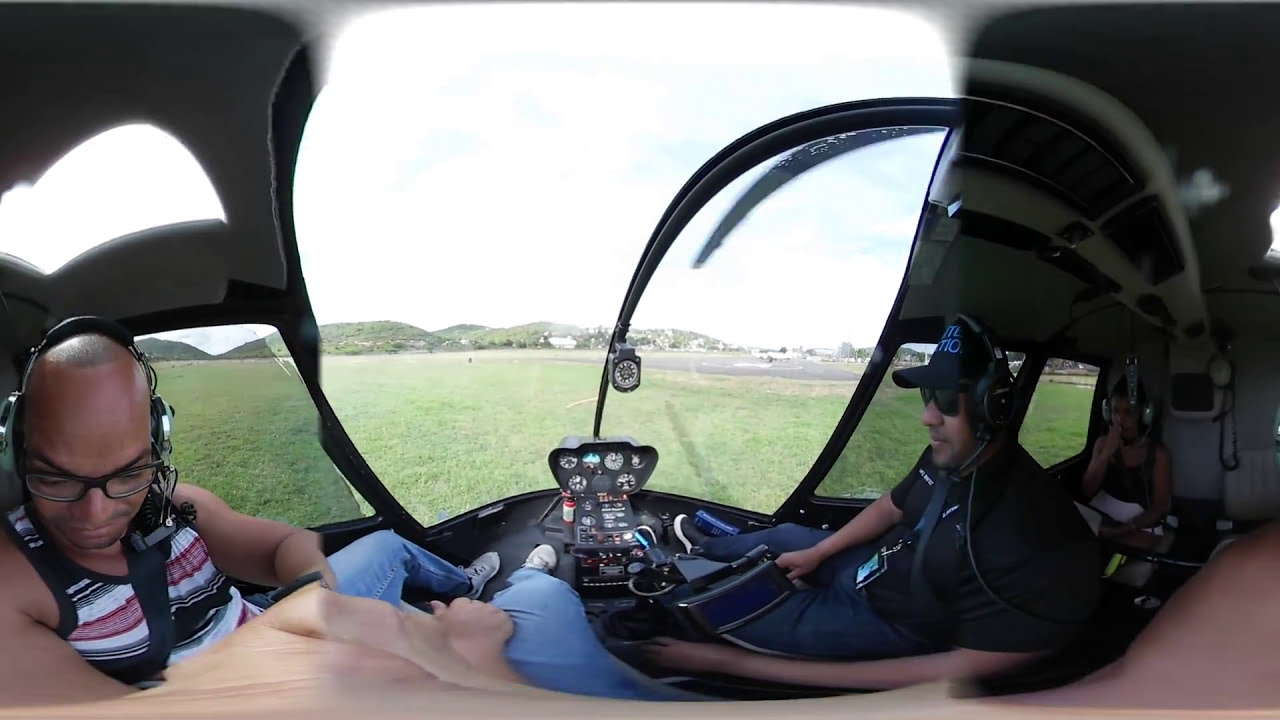This detailed image depicts the interior of a helicopter cockpit with a slight lens distortion affecting the orientation. In the bottom center, the cockpit control panel is visible, featuring a small cluster of instruments including four on the top, three on the bottom, and several small indicator lights in the middle. The helicopter is slightly above the ground, situated in a grassy area near a tarmac, with large grassy hills and a bright, cloudy sky in the background.

Two men with dark brown skin, possibly South Asian, sit in the foreground of the image. Both are wearing headsets and glasses. The man on the right, presumed to be the pilot, is wearing a black baseball cap with blue writing, dark sunglasses, a black short-sleeved t-shirt, dark blue jeans, and a lanyard with a badge around his neck. He has his right hand on the control stick positioned between his legs. The man on the left is bald and wearing a black, white, and red-striped tank top, lighter blue jeans, and white tennis shoes. He has glasses with clear lenses. Both men are secured with seat belts.

Additionally, a third person is visible in the background, sitting to the right and turned around, engaging with the other two men. The helicopter's side is open, suggesting an open or missing door. The scene outside the helicopter adds an expansive feel to the image, showcasing its position ready for takeoff.